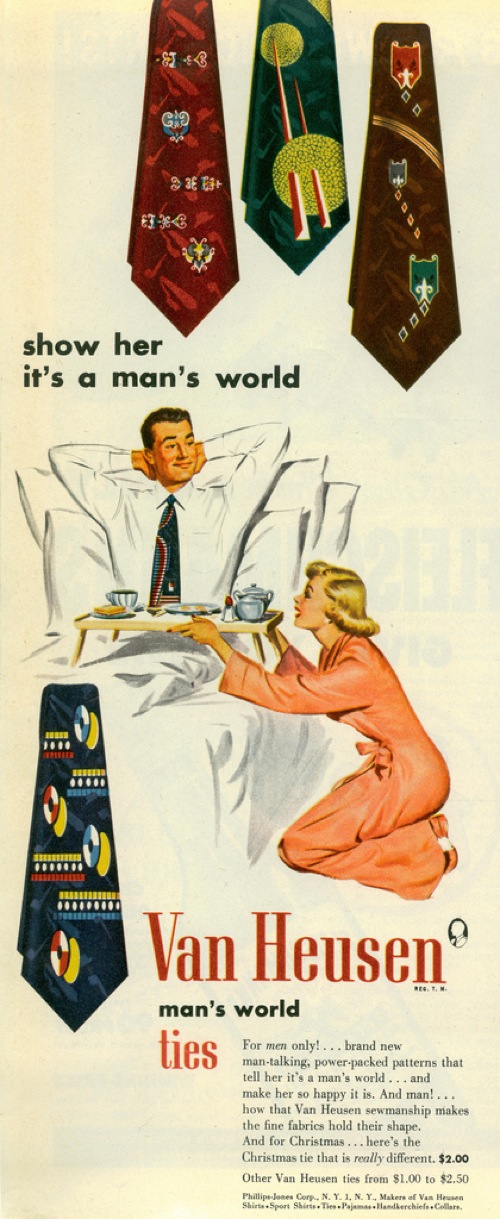This vintage advertisement for Van Heusen Ties prominently features a scene depicting a man lounging in bed, propped up against pillows with a smug expression, his arms comfortably behind his head. Dressed in a white long-sleeved button-down shirt and a tie, he appears relaxed and content. Beside him, a stereotypical 40s or 50s housewife with curled blonde hair and a long orange dress or robe kneels on the floor, presenting him with a breakfast tray laden with a plate, mug, and coffee pot.

At the top of the ad, three ties are showcased against a yellow or beige-yellow background: two dark red ties and one dark blue or green tie featuring abstract circular designs. The headline boldly reads "Show her it's a man's world," reinforcing the era's cultural norms. Below the main image of the man and woman, there’s another tie displayed with the text "Van Heusen Man's World Ties." Additional smaller text notes that the ties are priced from $1 to $2.50, emphasizing the appeal and affordability of the brand.